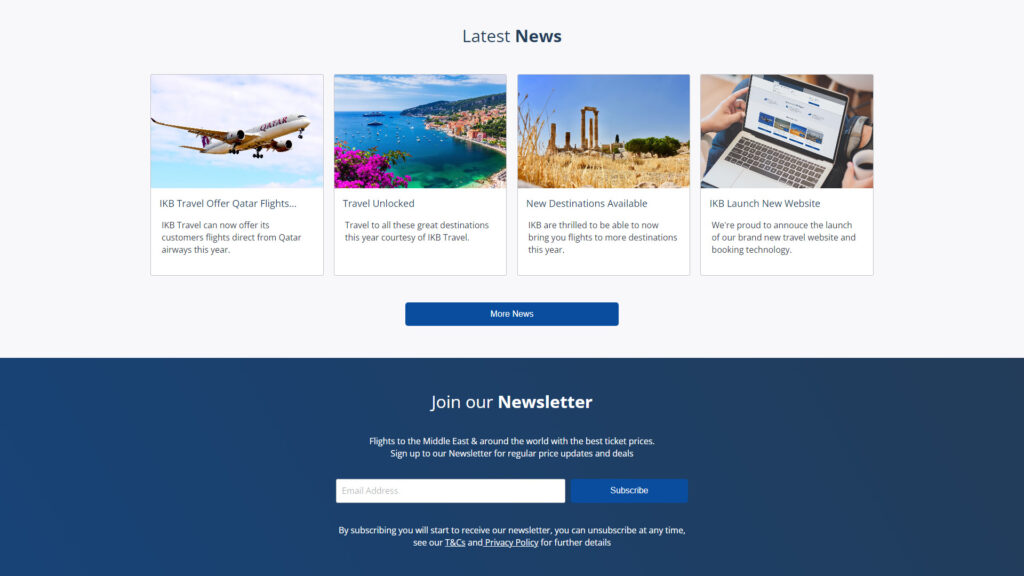The image represents a webpage with a layout that is about twice as wide as it is tall. The background of this webpage is a light gray color, covering approximately the top two-thirds of the image. 

At the top-center of the webpage, there is a header composed of dark blue text that reads "Latest" followed by a bold, dark blue "News", with the "L" and "N" capitalized.

Below the header, there are four images aligned horizontally and centered. Each image includes a headline and a brief paragraph. The first image depicts an airplane with the caption "IKB Travel Offers Qatar Flights" and a paragraph beneath it. The second image shows a tropical beach scene, accompanied by the caption "Travel Unlocked" and a descriptive paragraph. The third image features ancient ruins in a desert, with the caption "New Destinations Available" and an accompanying paragraph. The fourth image provides a top-down view of a person using a laptop, captioned "IKB Launch New Website" with its corresponding paragraph below.

At the bottom of the light gray area, there is a centered blue button labeled "More News" in white font.